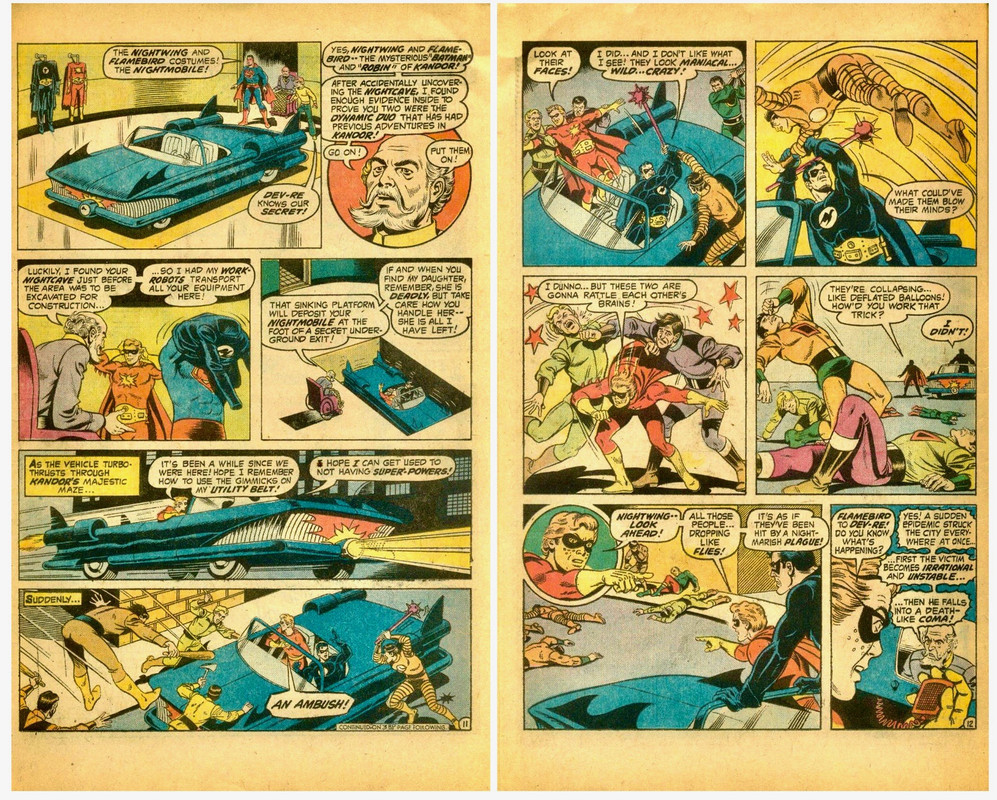This image showcases two pages from an aged, yellowed comic book, likely indicating its vintage nature. Each page contains six frames, vividly colored but predominantly yellow due to aging. The comic features various superheroes, including Batman, Robin, Superman, and characters dressed as Nightwing and Flamebird. A blue Batmobile is prominently depicted in the upper left-hand corner with Batman and Robin beside it. Dialogue bubbles, such as "Devray knows our secret" and dramatic statements about faces looking "maniacal, wild, crazy," add to the narrative tension. One superhero brandishes a bird emblem on their chest. The edges of the pages appear frayed, further emphasizing the comic's old age and historic value.